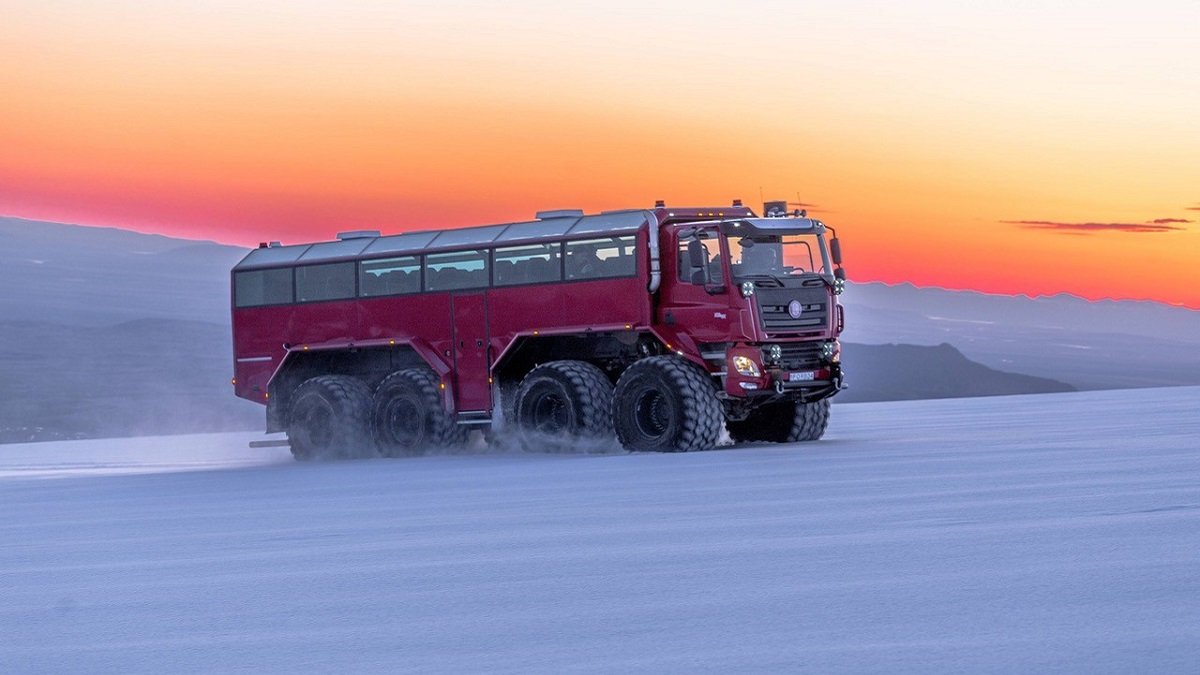This photograph captures a desolate, snowy landscape with a rugged, heavy-duty vehicle at its center. The large, dark-red vehicle, reminiscent of a school bus, features eight tires—four on each side—and is equipped with windows both along its sides and on top, akin to an observation car on a train. The vehicle is driving up a snowy incline, with snow spraying from its tires, highlighting its movement. The front end has a black grille and yellow lights shining out, while two white circles are visible on the roof towards the back. The sky above transitions from a deep red near the horizon, to orange, and finally to a cream color at the top, suggesting either a sunrise or sunset. In the background, light-blue snowy hills add to the stark, wintry atmosphere.